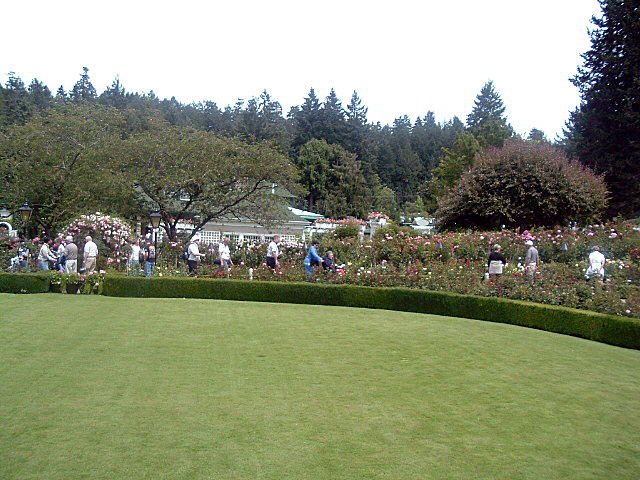The color photograph captures an outdoor scene featuring a large, flat expanse of grass that resembles a putting green, surrounded by a neatly trimmed rectangular hedge. Beyond this hedge lies a vibrant garden filled with an array of wildflowers. Approximately 12 to 15 people, mostly older individuals dressed in khakis and polo shirts, are seen walking around or standing within the flower garden, suggesting a casual stroll rather than any form of gardening or fruit picking. The backdrop of the image features a white building with a gray roof, enveloped by lush green trees including pine trees, and topped by a white sky, enhancing the serene and picturesque setting.